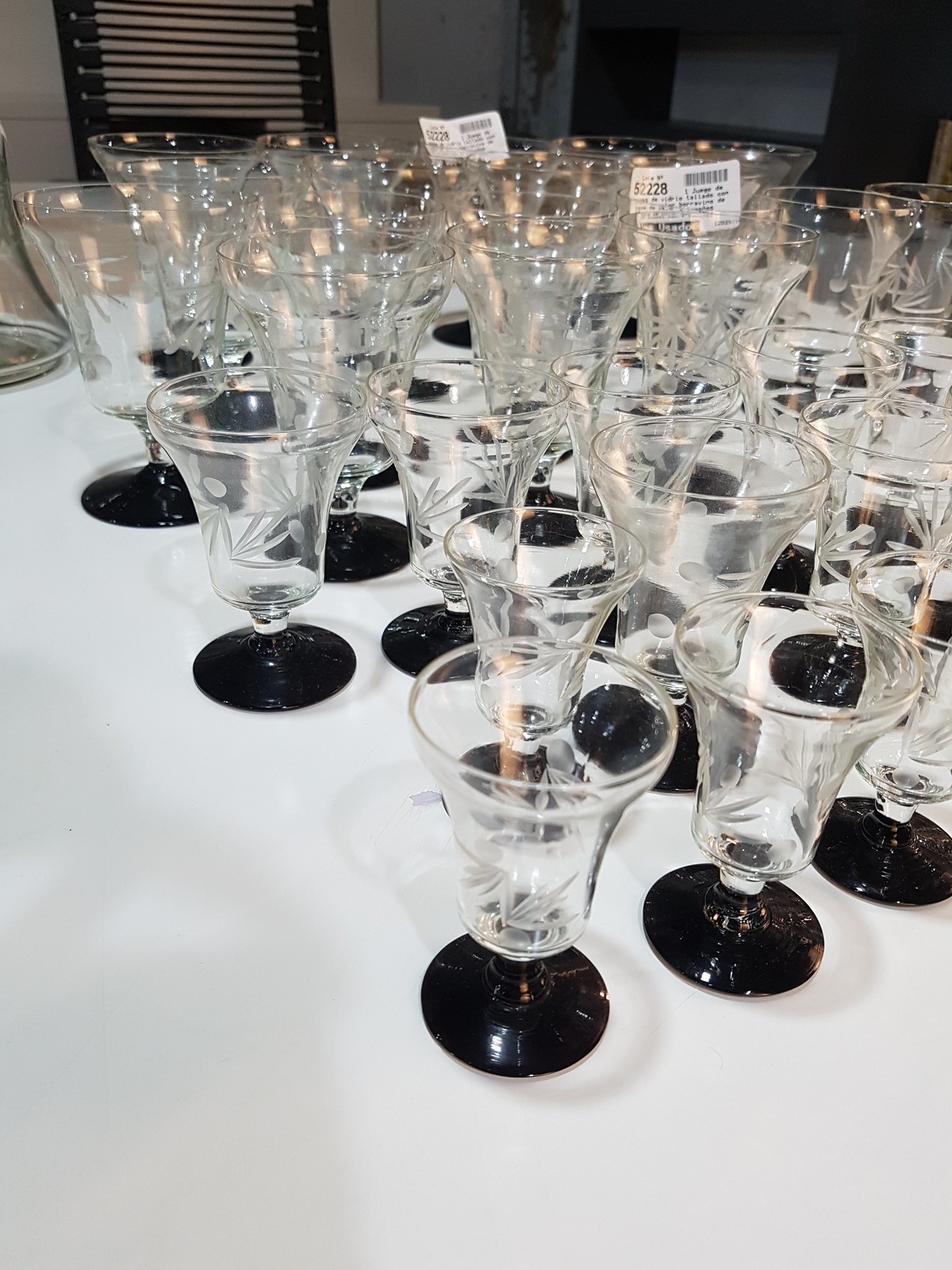The image features a large collection of approximately 25 to 30 crystal goblets, neatly arranged on a white tablecloth or countertop, which serves as the backdrop. These goblets, each with a black cylindrical pedestal stem, transition into clear, etched crystal bodies adorned with intricate patterns resembling thin leaves and circles. The goblets are wider at the top and taper down to the base, allowing more liquid to be held in the upper part. In the far right corner of the photo, one goblet displays a white sticker with numbers and a barcode. A similar sticker can be found on another goblet, indicating a retail setting. The background reveals faint shadows on white walls, and in the far left corner, partial visibility of a window with white lines can be observed. This close-up, portrait-oriented image emphasizes the intricate design and arrangement of the goblets, filling almost the entire frame.